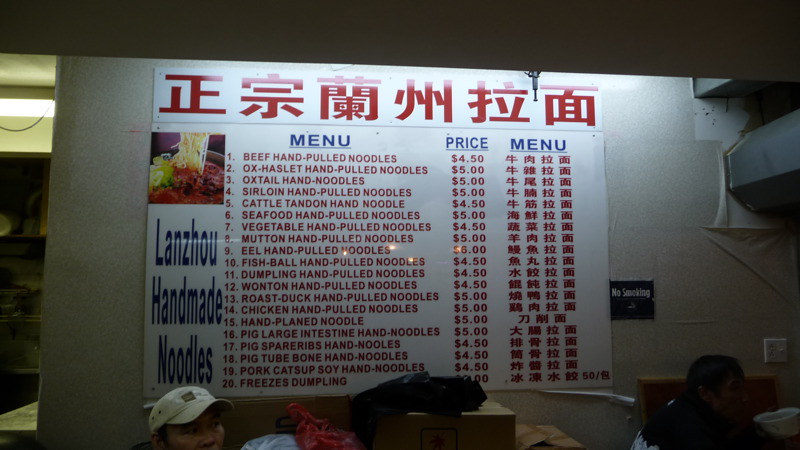This image captures the extensive menu of an Asian restaurant, with the exact cuisine unspecified. Dominating the left side of the menu, the bold heading “Lanzao Handmade Noodles” suggests the restaurant’s specialty. Along the top, Asian alphabetical characters are prominently displayed, though the exact language is unclear.

Above the text, a tempting image showcases a bowl of what seems to be a hearty soup, with noodles being elegantly lifted out, hinting at a deliciously comforting meal reminiscent of pho, though there is no direct mention of it.

The menu is structured with three main columns: the first column lists menu items in English, the center column presents the prices, and the third column features names written in Eastern characters. Menu and price headers are highlighted in bold blue at the top.

The variety of noodle dishes is notable, with nearly every item including the word “noodles.” Offerings range from “Beef Hand Pulled Noodles” to more exotic options like “Eel Hand Pulled Noodles” and “Ox Haslet Hand Pulled Noodles.” Other dishes include “Sirloin Hand Pulled Noodles,” “Seafood Hand Pulled Noodles,” and unique entries like “Pick Large Intestine Hand Noodles.” Dumplings and wontons also make an appearance, showcasing the menu's diversity.

Pricing is straightforward, mostly between $4.50 and $5. The price of one dumpling dish is obscured by a customer wearing a ball cap, who stands in front of the lower part of the menu, which is mounted on a wall. 

In the background, a bright overhead light illuminates another room to the left, while a “No Smoking” sign is clearly visible to the right. An overhead light specifically highlights the menu, drawing attention to its expansive selection. The atmosphere suggests a casual, inviting dining experience with a focus on traditional, handcrafted noodle dishes.